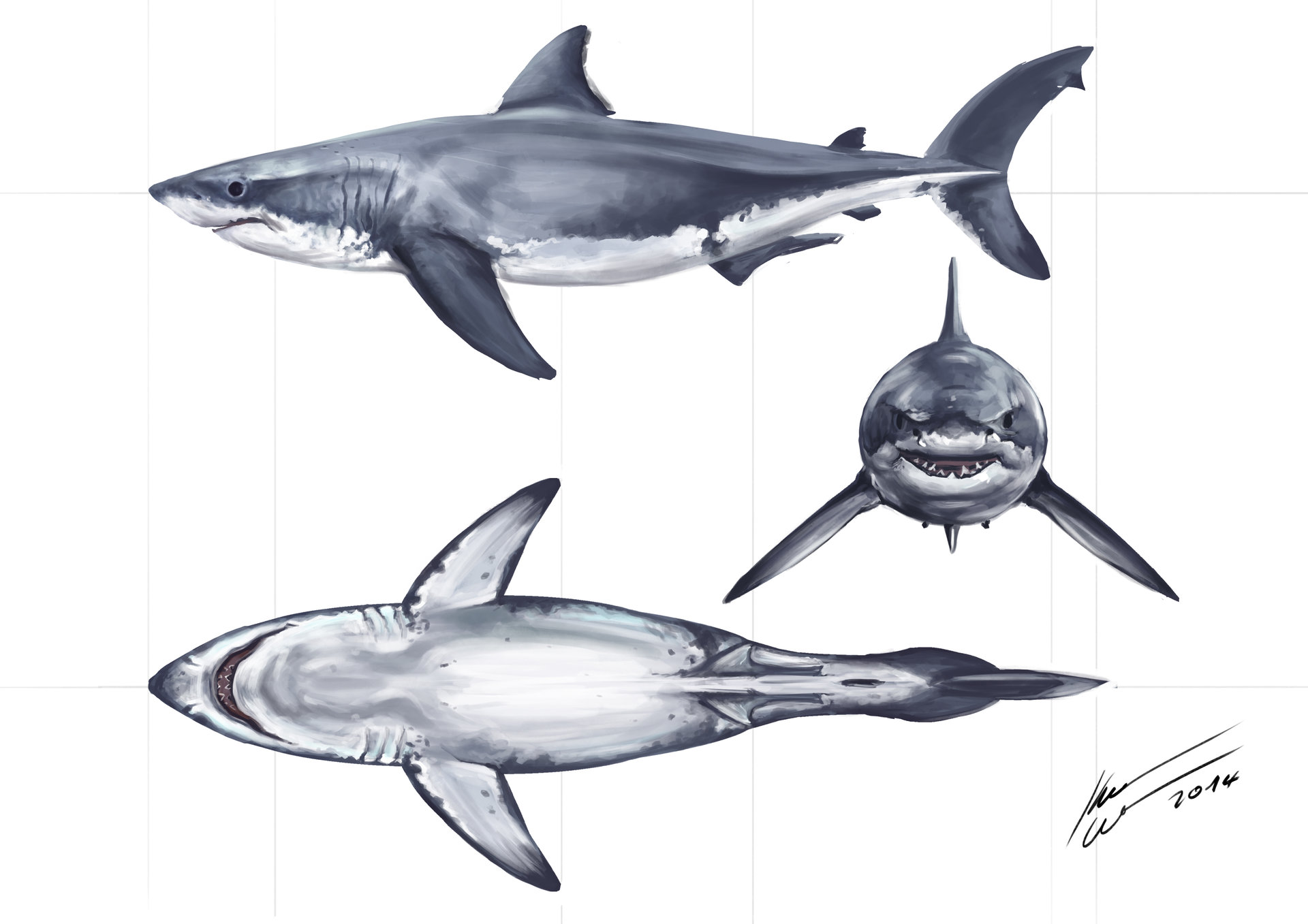In this image, we see a detailed watercolor sketch of a typical large oceanic shark, displayed on a white background paper that features faint horizontal and vertical lines, resembling a diagram sheet. The illustration showcases the shark from three different perspectives. At the topmost position, there is a side view of the shark, showing its full length with the head on the left and the tail on the right, highlighting its gray upper body and white underbelly. Below this, towards the right, is a front view of the shark swimming towards us, with its mouth open to expose sharp teeth, and outlined are the eyes and side fins. The bottommost illustration depicts the shark from beneath, focusing on its white belly and the underside features. In the bottom right corner of the image, we can see the artist’s signature in black, accompanied by the year 2024.